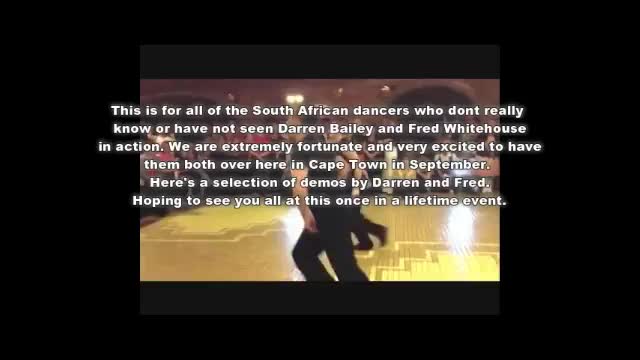The image features a black background with a black border, emphasizing a central scene where a crowd of people watches two men on a gym-like hard floor, reminiscent of a dance stage. The crowd appears captivated by the two men, identified as Darren Bailey and Fred Whitehouse, who are prominently positioned in the scene. Superimposed over the image is white text that reads: "This is for all of the South African dancers who don't really know or have not seen Darren Bailey and Fred Whitehouse in action. We are extremely fortunate and very excited to have them both over here in Cape Town in September. Here is a selection of demos by Darren and Fred, hoping to see you all at this once-in-a-lifetime event." The image features a range of colors including black, white, brown, yellow, tan, gray, and red, contributing to the vibrant and inviting atmosphere that serves as an invitation to an eagerly anticipated dance event.